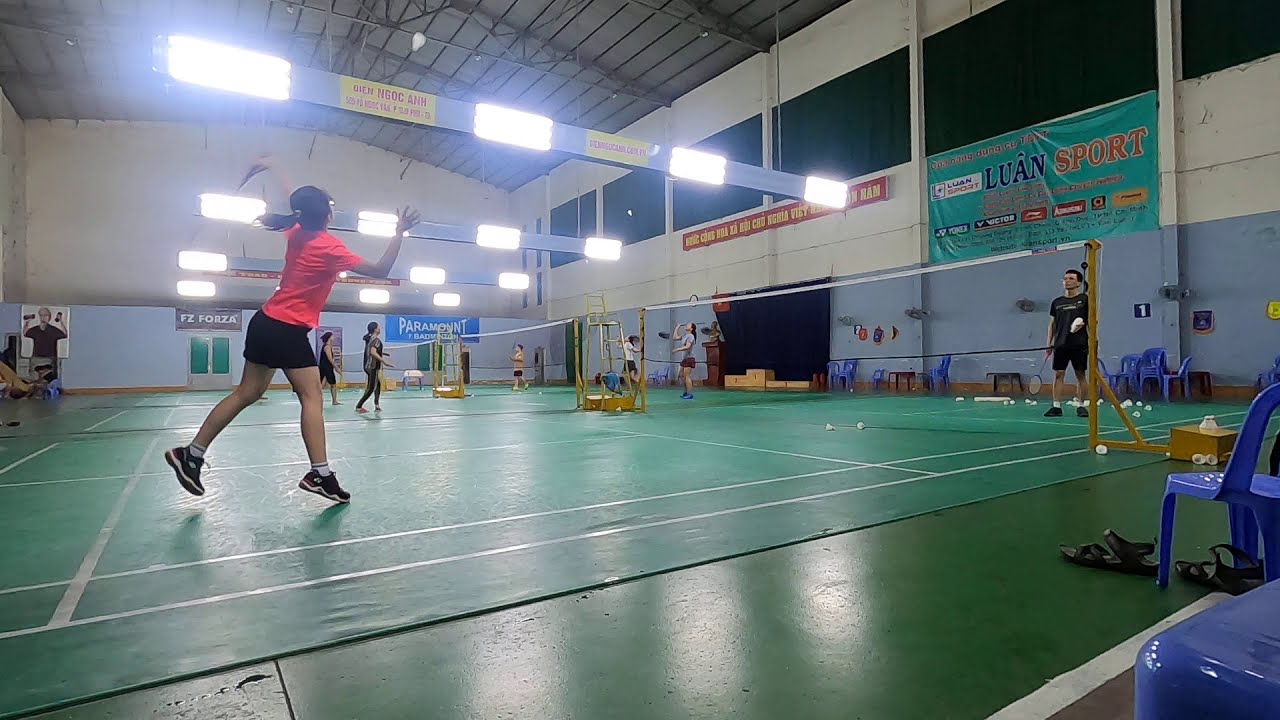In an expansive, warehouse-style gymnasium with an arched roof and intense lighting, multiple people are engaged in a lively game of badminton. The gym's floor is painted green, overlaid with green and white striped mats. There are two courts, each equipped with a net. Bright blue plastic chairs are arranged along the sidelines, with black strap shoes notably placed by one of the chairs. The walls are painted white on the top half and light blue on the bottom, adorned with various banners and posters, including ones that say "Luan Sport," "Paramount," and "FC Forza." In the forefront of the image, a girl with a ponytail under her hat, donned in an orange shirt, black shorts, and tennis shoes, is actively hitting a shuttlecock. Her opponent, dressed in a black shirt and black shorts, stands ready on the opposite side. In the background, several other pairs can be seen playing badminton, while someone is lifting weights further away. Spectator areas are visible above the courts, suggesting a well-structured and organized sports facility.